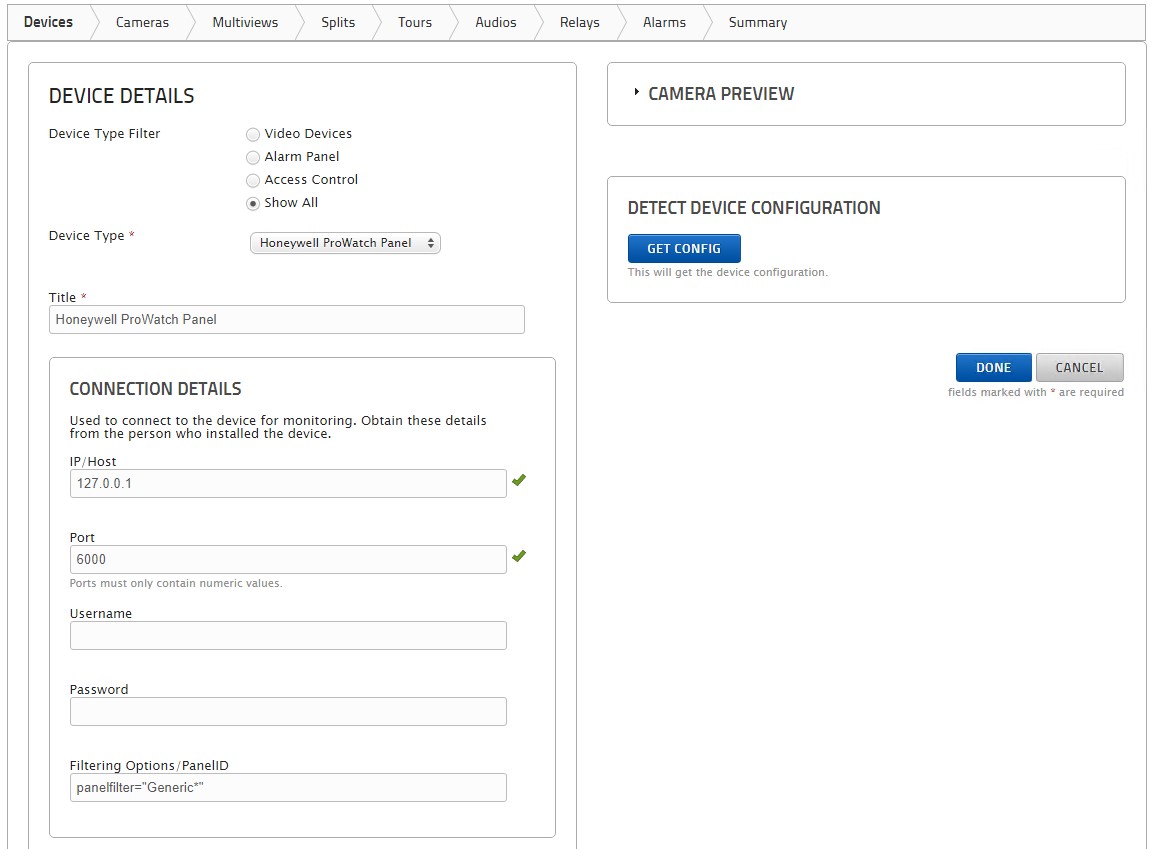The image is a screenshot of a user interface, likely for a router or a home security system. The background is predominantly white with thin black lines delineating various sections, and all text is in black. The monochromatic layout is interrupted only by a couple of blue clickable buttons on the right-hand side. At the top of the interface, there are several navigation tabs labeled: "Devices," "Cameras," "Multi-View," "Splits," "Tours," "Audios," "Relays," "Alarms," and "Summary." The current view is on the "Devices" tab, which opens up to the "Device Details" section. Here, there is an option to filter device types, and "Honeywell ProWatch Panel" has been selected. The connection details such as IP address, port, and filtering options are displayed below, though the username and password fields are left blank. On the right side, there is a section labeled "Camera Preview," suggesting functionality for controlling a home security system. Below that, there is a blue button labeled "Detect Device Configuration" for fetching the configuration settings, and two additional buttons: a blue "Done" button to finalize changes and a gray "Cancel" button to discard any actions.